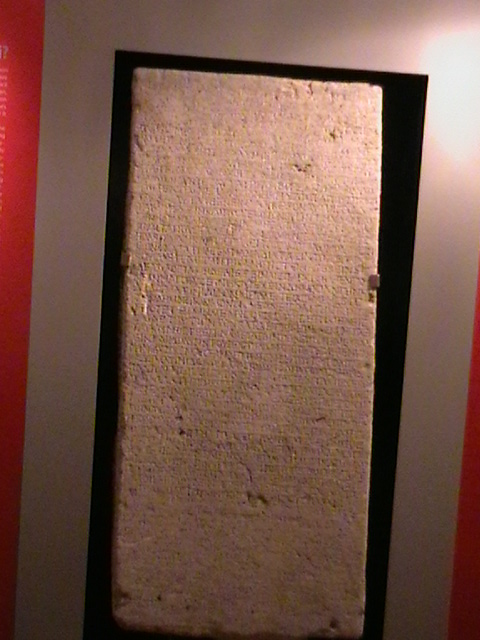The photograph shows a rectangular stone tablet with ancient writing etched into it, possibly cuneiform or Roman in nature. The greyish, slightly worn tablet is haphazardly positioned in the frame, giving the image a skewed, diagonal appearance. Mounted against a black background and framed by a white backing, the tablet is on display, likely in a museum or gallery. The contrasting colors—black, white, and red stripes on either side—enhance the visibility of the tablet. Despite a few pits and marks indicating its advanced age, the stone remains in remarkably good condition, with only minor damage at the bottom. The writing on the tablet is uniform and neatly carved, although unreadable from the photograph, suggesting it was crafted with precision using tools like a pick and hammer. The overall scene needs some adjustment, possibly photoshopping, to straighten the image.